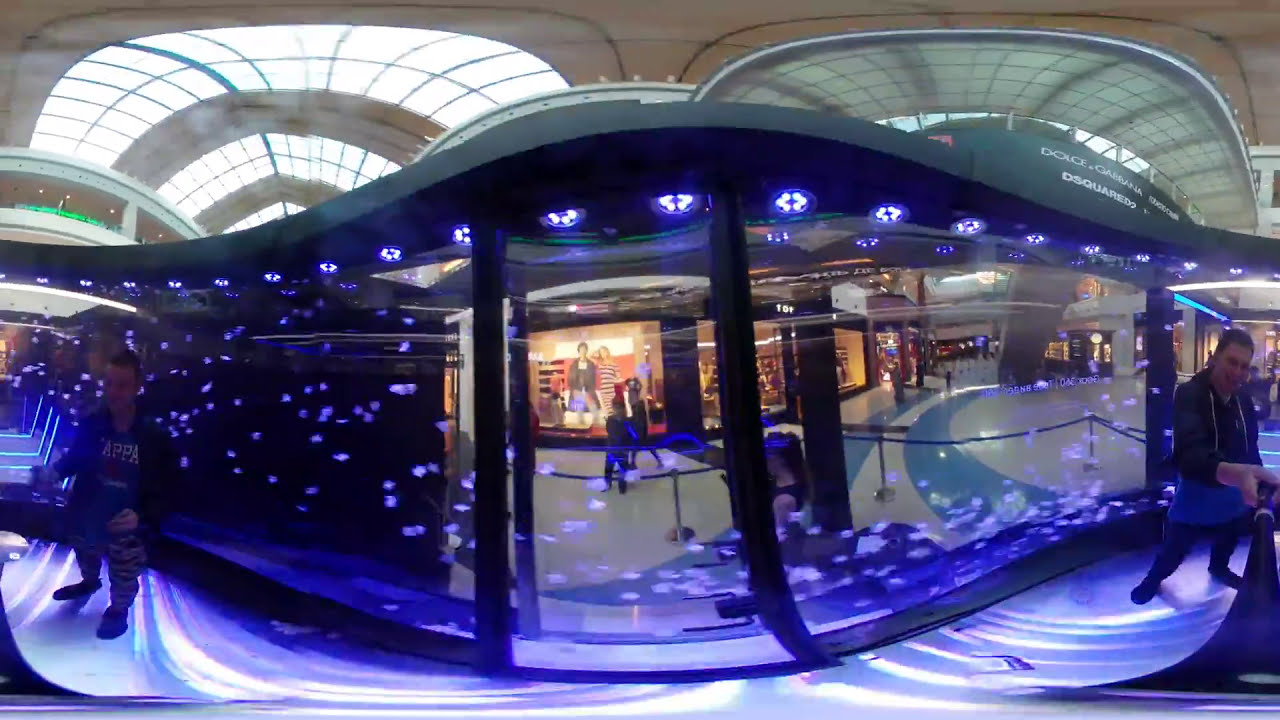The photograph depicts a spacious and vibrant area inside an indoor shopping mall, characterized by a large glass or plexiglass structure with striking lavender and purple lights on the walls, ceiling, and floor. The scene is bustling with activity; people can be seen standing near the illuminated enclosure, including a man in a black hoodie and dark pants using a selfie stick and another man in a dark jacket with a Kappa shirt and camouflaged pants.

The background reveals various storefronts with mannequins displaying fashion, notable among them is a Dolce & Gabbana store. The floor features a white surface with prominent yellow and blue stripes. The mall has a high ceiling with glass skylights that allow daylight to filter in, creating a bright and lively atmosphere. There is visible advertising for clothing, and the layout includes higher levels and a stairway, suggesting a multi-tiered shopping experience.

This detailed setting offers a glimpse into a modern, well-lit shopping hub showcasing luxury brands and contemporary decor, framed perfectly by the architectural transparency and dynamic lighting of the glass enclosure.